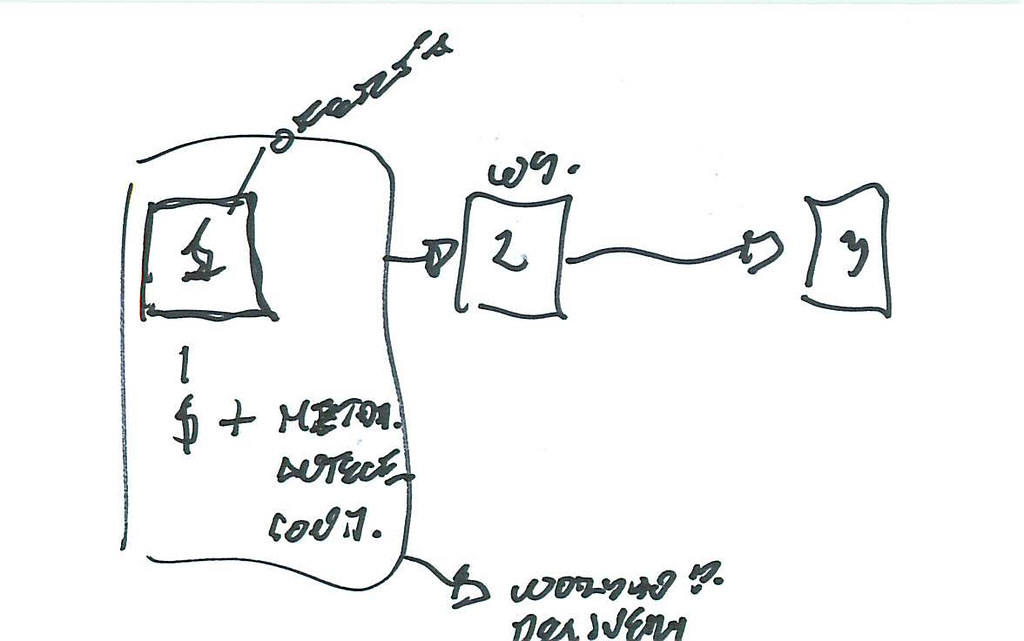The image displays a hand-drawn set of notes on a white surface, resembling a photocopy due to its presentation. The notes contain three primary boxes. The largest box encompasses another smaller box within it. Inside the smaller box, there is a number "1", accompanied by an indiscernible scribble adjacent to a line. Beneath the "1", a note reads "1 $ +", followed by illegible text due to the poor penmanship.

An arrow extends from the largest box to the right, pointing to more unclear text, with the bottom word partially cut off as if from a photocopy. To the right of the large box, a line leads to a boxed arrow that points to another boxed number "2". Above this box, the notation "WS." is visible. Additionally, there is a poorly drawn squiggly line with an arrow, which connects to a squiggly, irregularly shaped box containing the number "3".

Overall, the notes are difficult to decipher due to poor handwriting and incomplete text, giving them a rough and unrefined appearance.